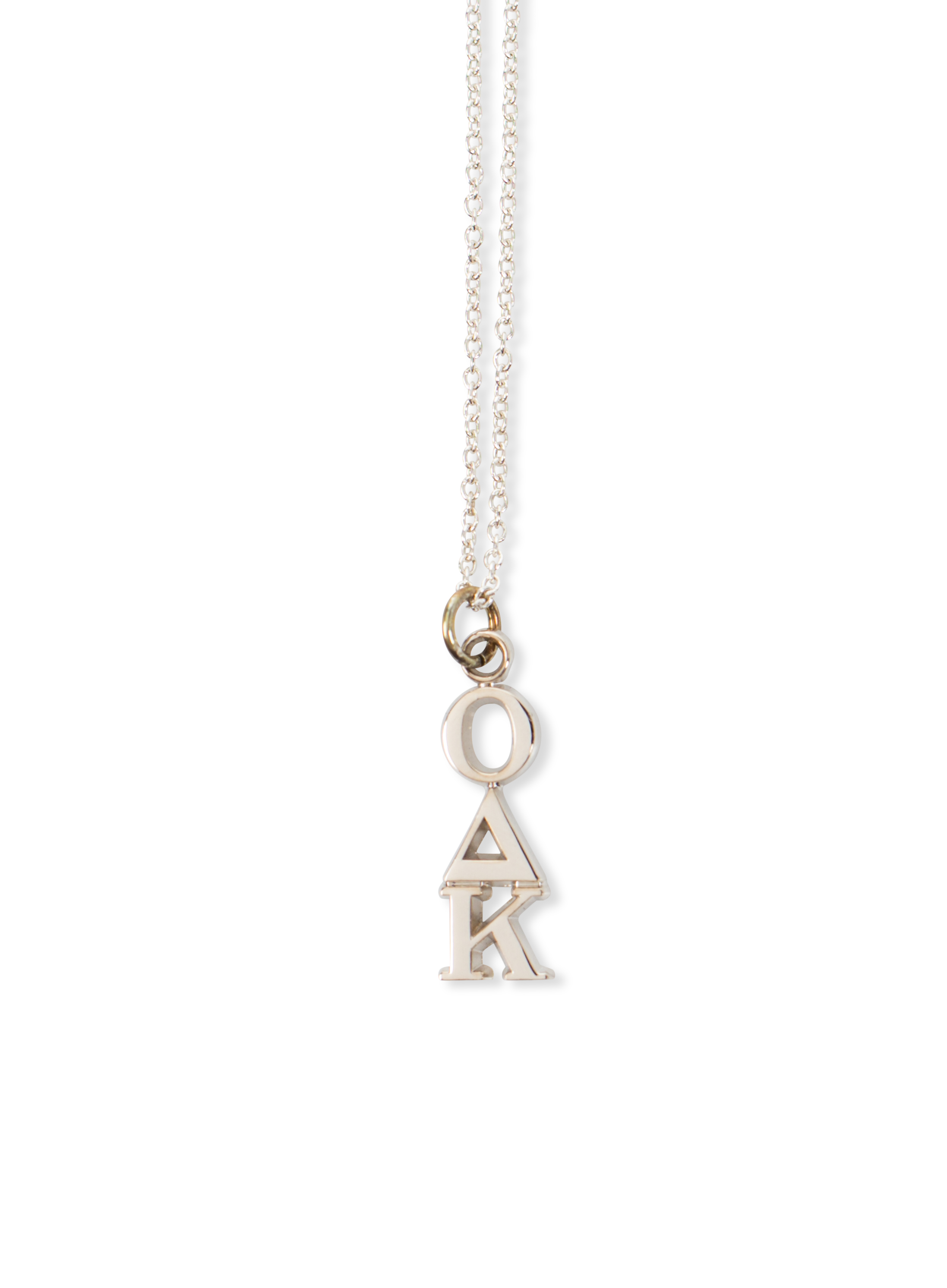The image displays a necklace set against a plain white background, with subtle shadows cast to the right of the chain. The necklace features a chain composed of very fine, interlinked loops that appear light gold in color. It descends from the top of the image and circles around a deeper gold-colored loop. Attached to this main loop is a smaller gold loop, from which hangs a vertical sequence of three characters - "O", a triangle with an open center resembling an "A", and "K". Together, these characters spell out "OAK". The craftsmanship of the chain appears delicate yet sturdy, suggesting a well-made and casual piece of jewelry.